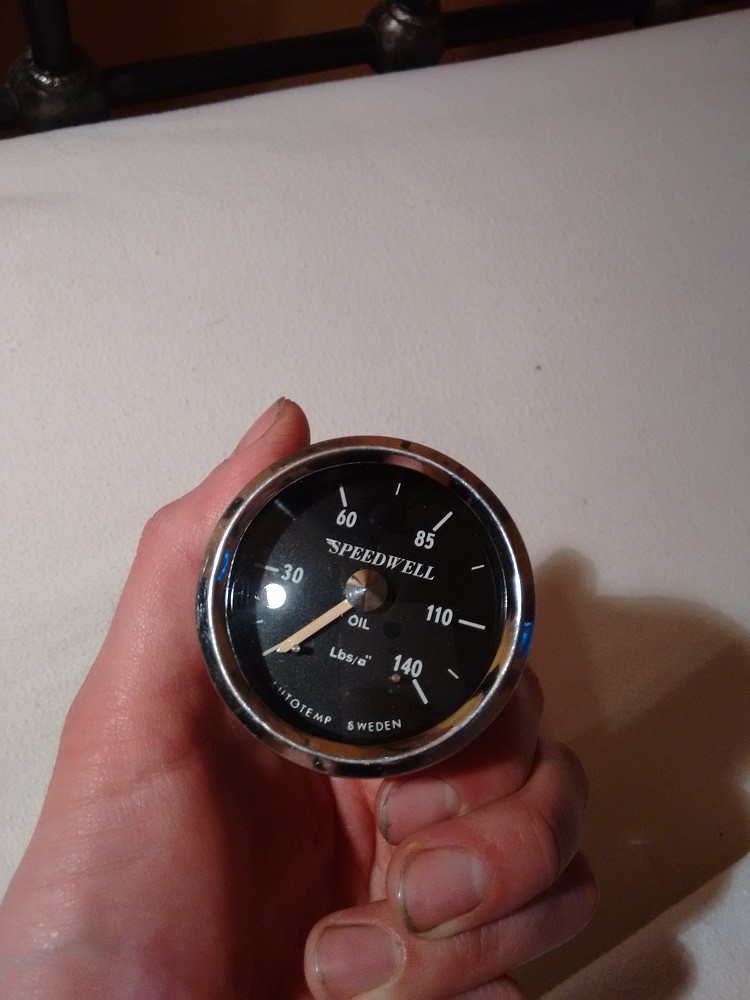In this rectangular photograph, we see a close-up shot of a white countertop or table, with a dark background partially visible in the upper left corner. The focal point of the image is a man's hand, which enters the frame from the lower left corner. His palm is facing up, and his thumb and fingers are gripping a round instrument that resembles a speedometer. The item is rimmed with a tortoise-shell-like color, featuring a black face with white markings.

The numbers displayed on the instrument range clockwise from 30 to 140, clearly marked at intervals of 30, 60, 85, 110, and 140. At the center of the face, where the single hand of the gauge points to the lower left, the brand name "SPEEDWELL" is prominently written in all-capital white letters. Just below that, the word "OIL" appears, followed by the abbreviation "LBS/A," likely indicating measurements in pounds. In the lower part of the instrument's face, the word "TEMP" and "SWEDEN" are also printed in white.

The man's fingernails are notably dirty, with what appears to be oil or grime embedded beneath them, highlighting that the fingernails are short but heavily soiled. This adds a rough, working-man quality to the image, emphasizing the hand's likely involvement in mechanical or labor-intensive tasks.